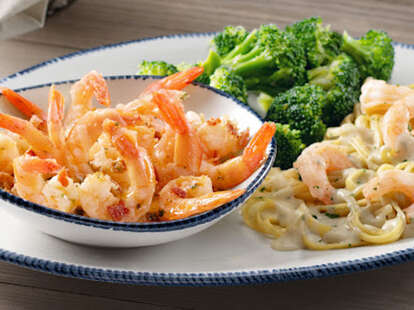The image showcases a restaurant dish consisting of a bowl of sautéed shrimp, shrimp Alfredo pasta, and broccoli, all served on a coordinating white plate with a blue edge, matching the bowl. The sautéed shrimp in the bowl on the left is garnished with a sauce, possibly butter. To the right of the bowl, the creamy Alfredo pasta, featuring more shrimp, is presented with a light yellow hue. Above the pasta, fresh broccoli florets add a vibrant green contrast, appearing lightly coated in butter. The dish is arranged on a countertop, making it look like an appealing item for a restaurant advertisement. The shrimp and broccoli stand out as the most noticeable elements, with the dish and bowl's blue-edged design unifying the presentation.